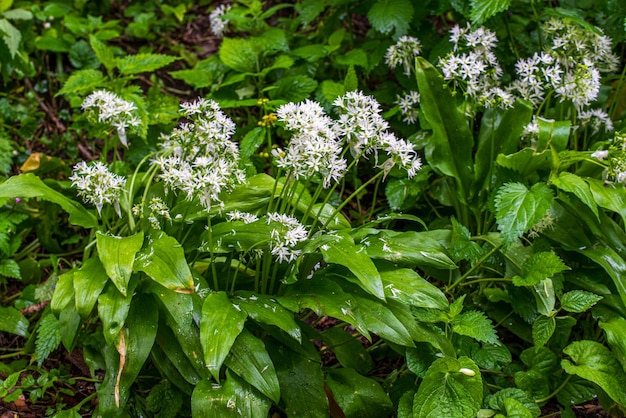This is a horizontal color photograph capturing a natural garden or forest scene. Dominating the upper right-hand corner and extending across roughly 80% of the frame, clusters of delicate, tiny white flowers with pointed petals emerge at the end of thin stems. These flowers resemble small daisies and are in bunches, growing amidst a rich array of foliage. The scene showcases a mix of about four or five different types of plants, including very large green leaves, possibly of tropical origin. Amongst the foliage are nettle-like leaves, adding to the diverse, possibly wild, and unmanicured appearance of the setting.

The lower right-hand corner features prominent large leaves that could be from other plant species, further enhancing the impression of a natural, untended environment. The ground beneath is visible, covered with a layer of leaves, twigs, and soil, indicative of a forest floor where organic material has been decomposing. In the background, additional green plants and what looks like ivy or vines contribute to the lush, verdant atmosphere. There is no text in the image, and the informal composition suggests that it is likely a snapshot rather than a professionally styled photograph.